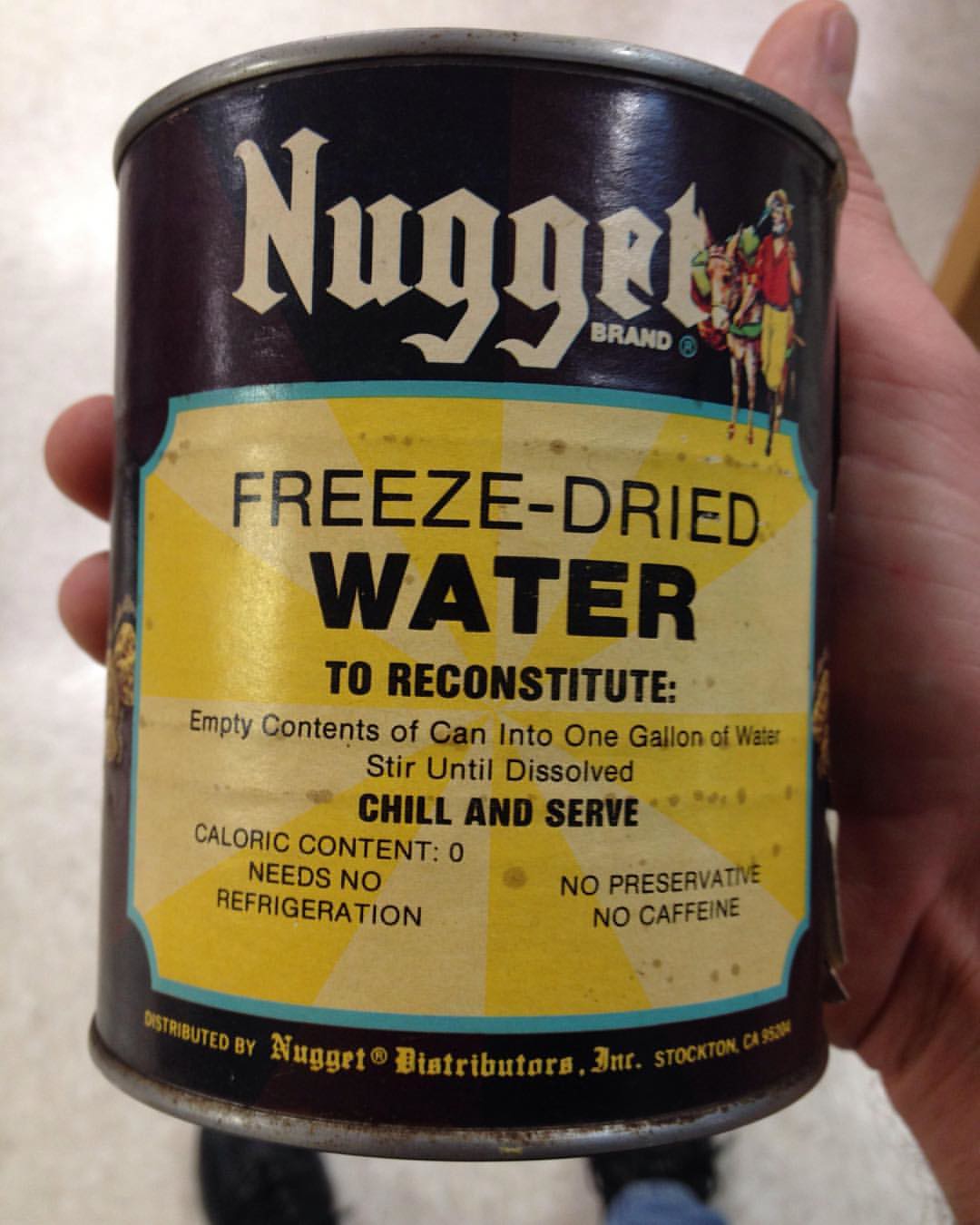A right hand is featured in this image, showing the wrist, part of the palm, the thumb, and the tips of two fingers. The hand is gripping a large can with a black label. The label prominently displays "Nugget Brand" in white letters at the top. Below the brand name is an illustration of a man in a hat walking beside a donkey. There is also a light yellow emblem resembling the sun, with darker yellow rays emanating from it. The yellow label includes detailed text explaining that this is "freeze dried water"; to prepare, one must empty the contents of the can into one gallon of water, stir until dissolved, chill, and then serve. Additional information on the label mentions that the product has zero caloric content, requires no refrigeration, contains no preservatives, and is caffeine-free.